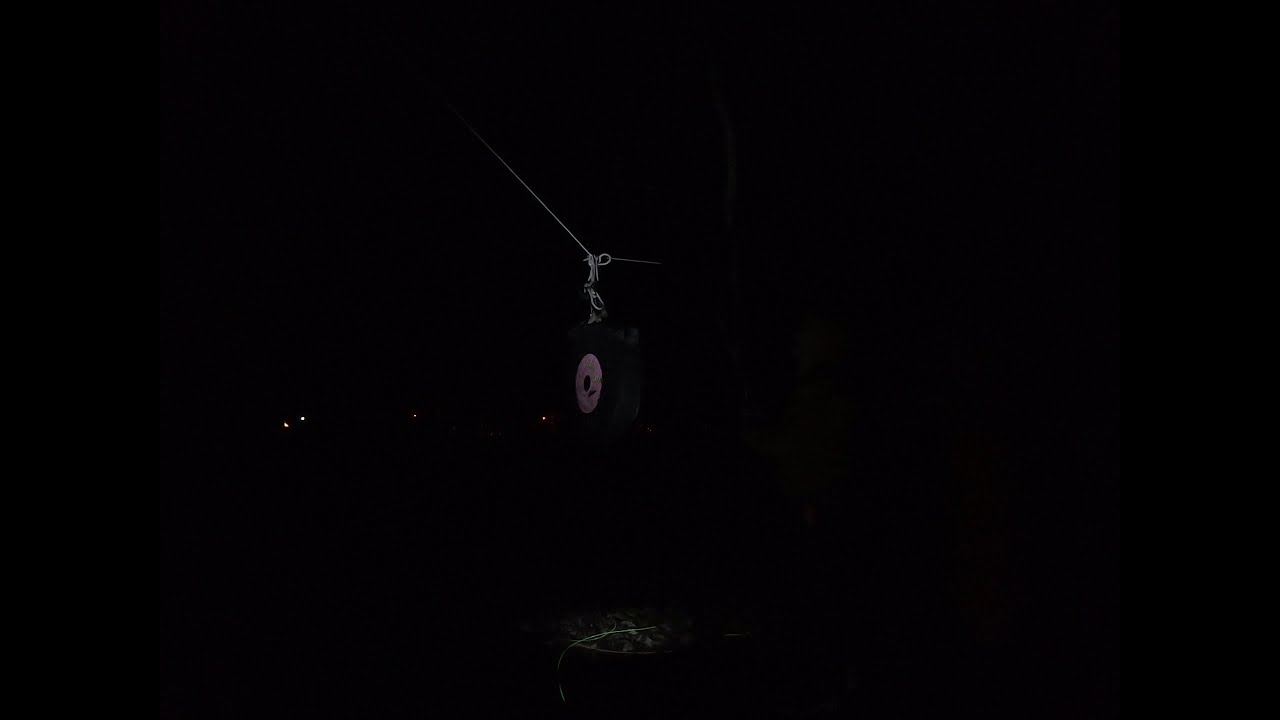The image is a landscape orientation color photograph taken at night, shrouded mostly in darkness. The scene appears almost entirely black, with around 98% of the background lacking discernible features. On the left side of the image, there are four small, bright white dots resembling distant lights. Towards the center, a faint, vertical silhouette is visible, potentially resembling a rope or clothesline, though its exact nature is unclear. Attached to this central element is a dark, indistinct object with a small pinkish circle on its side, though its details and edges are obscured by the surrounding blackness. On the right side, the image is entirely consumed by the dark, offering no further details. The photograph seems to capture a view from an interior space with a curtain partially pulled back, adding to the enigmatic quality of the scene. The overall style of the photograph leans towards representational realism, though the heavy darkness renders the scene ambiguous.